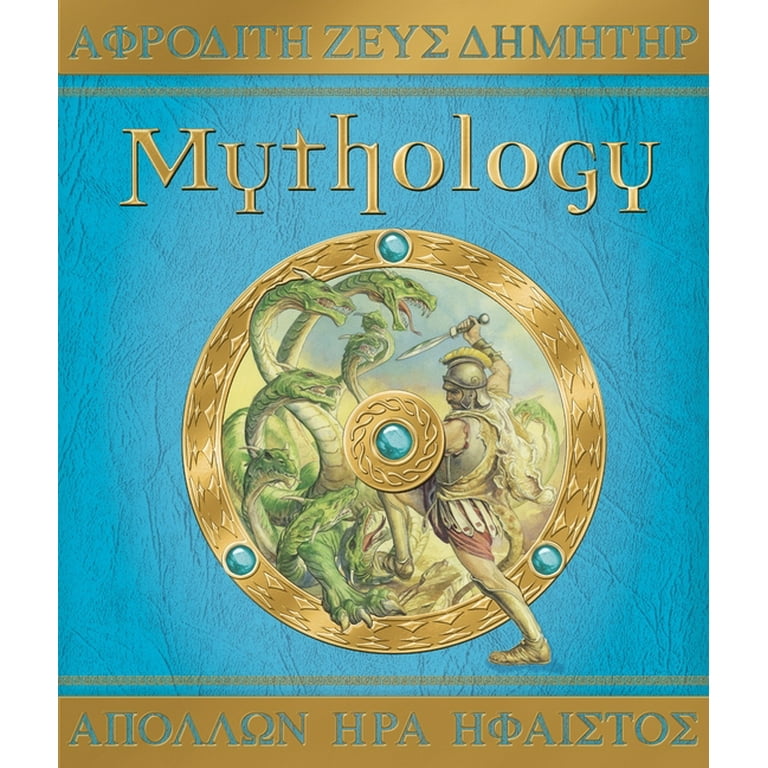The cover of an ancient-looking book, likely on Greek mythology, features a rich blue background with a texture resembling wrinkled fabric. At the top, in large, stylized gold letters, is the word "MYTHOLOGY." Surrounding the main illustration is a golden circle or medallion. This central image vividly depicts an intense battle between a heavily armored, silver-helmeted Roman soldier and a multi-headed dragon. The soldier, gripping a shield in his left hand and a dagger poised to strike in his right, is caught in mid-action, his back leg extending beyond the circle. His shield has a golden center with a teal accent. The dragon, a serpentine creature with numerous heads, is engaged in combat with the soldier. Surrounding the gold medallion are four small blue stones strategically placed at the top, left, right, and toward the bottom. Greek letters, including “HPA” in the middle, adorn the gold borders at the top and bottom. The bottom inscription, also in Greek script, adds to the authenticity and classical allure of the cover.